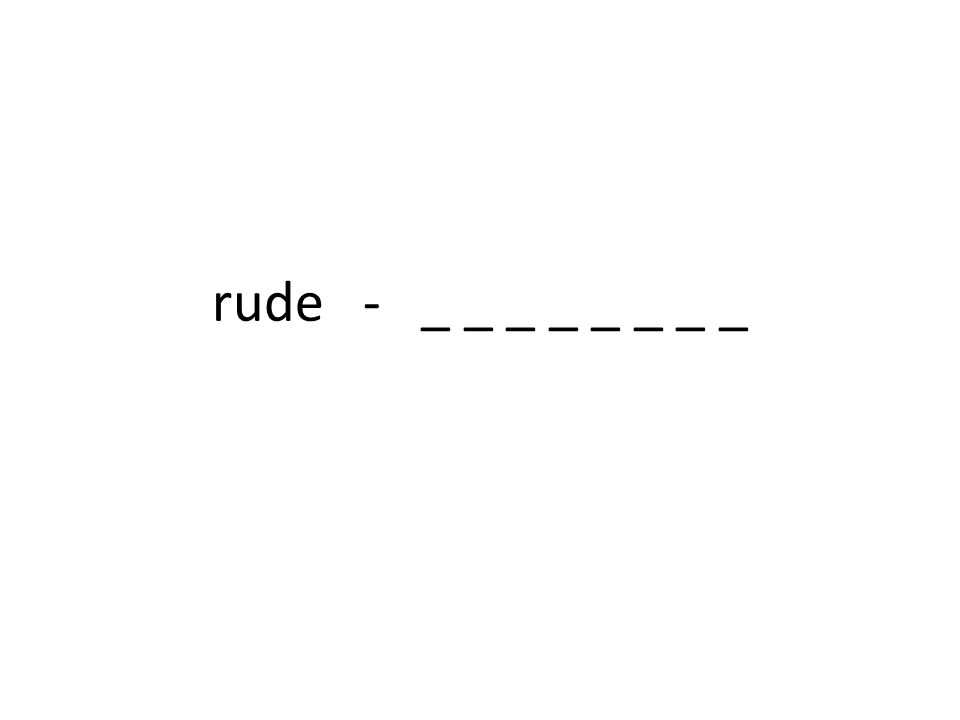This computer-generated image features a minimalist composition with a stark white background and black text. In the center of the image, the lowercase word "rude" is displayed, followed by a dash. Beneath the dash, there are eight black underlined spaces, suggesting a word-guessing game format, such as Hangman or Wheel of Fortune. The text is horizontally aligned and centered, with the empty spaces indicating that an eight-letter word should follow "rude." The simplicity and layout of the image evoke the style of a newspaper puzzle or a digital word game.